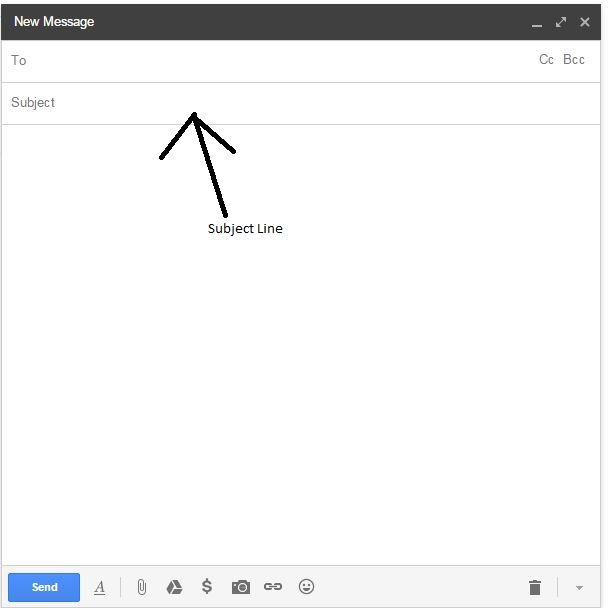The image depicts an email application's new message window. At the top of this window, there is a dark grey horizontal bar with the text "New Message" written in white on the left side. Below this bar, two input rows are visible. The first row contains the label "To" in dark grey on the left side, intended for entering the recipient's email address. Directly below this, the second row is labeled "Subject" in dark grey, with a thick black arrow pointing upwards into the subject input box, emphasizing the importance of this field. Additionally, underneath the arrow is the text "Subject Line" in black. Positioned towards the lower left part of the image, a blue rectangular "Send" button is present, with the word "Send" written in white across it. This button is clearly identifiable and positioned for easy access in the email composition window.